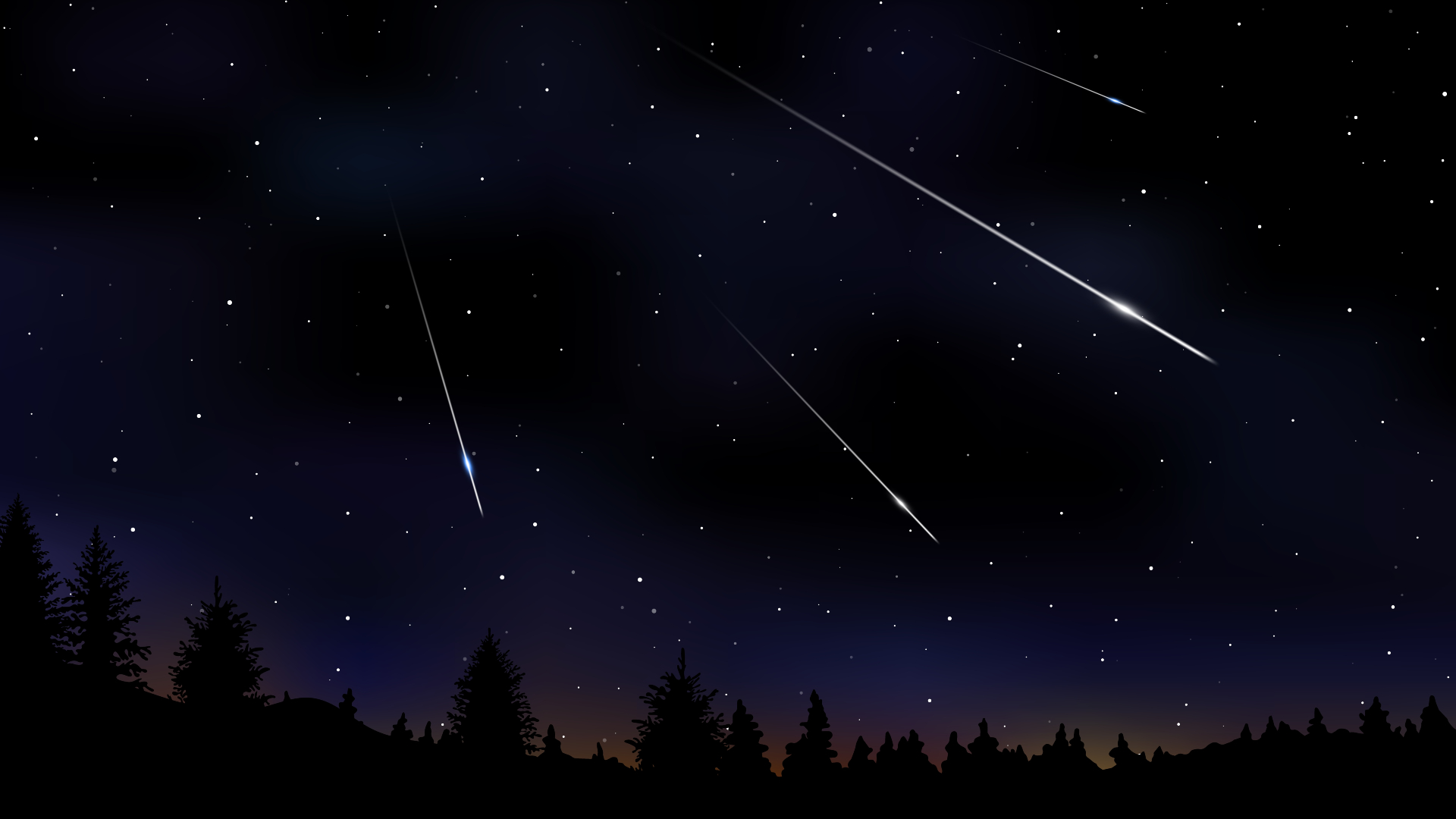This detailed image is an artistic rendition of a serene night sky, blending natural beauty with digital art. At the base, silhouetted pine or fir trees form a dark forest, contrasting with the sky above. The horizon starts with a subtle reddish or orange glow, gradually transitioning through shades of blue from light to dark. The sky is sprinkled with numerous sparkling white stars, evenly dispersed. Among them, four distinct shooting stars stand out, streaming diagonally from the left-hand side towards the bottom right. The first shooting star is small and short, located near the top right. The second, the longest, brightens significantly as it trails. The third is thinner and shorter, yet still features a bright tip. The last shooting star, larger than the third but smaller than the second, points almost straight down with a luminous tip. This striking image merges shades of black, navy, and a hint of purple, creating an enchanting night scene.